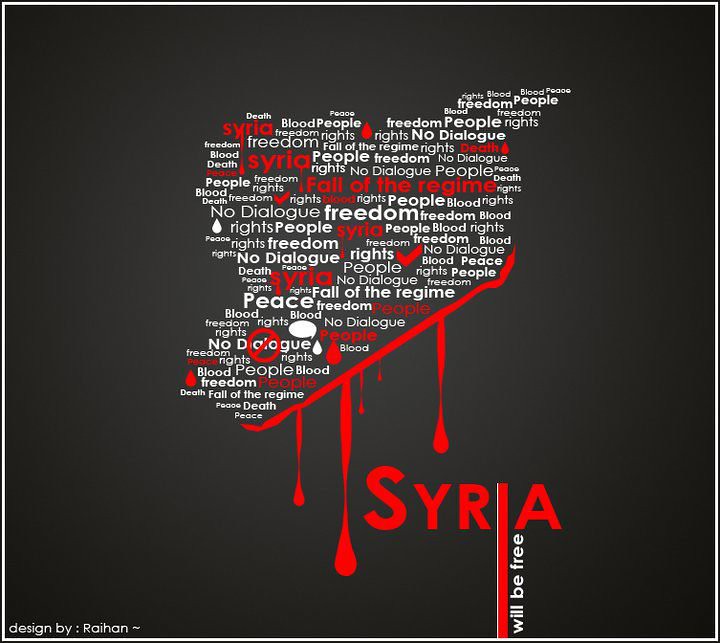The image features a prominent black background with an intricate design formed by multiple white words and phrases, such as "people," "freedom," "rights," "no dialogue," "death," and "blood." These words are repeatedly used to shape a central figure, which seems to represent the country of Syria. Interspersed among these words are impactful red highlights that include phrases like "Syria," "follow the regime," and "death," along with blood-red arrows and check marks. A striking red cross cuts through the words "no dialogue."

Toward the bottom of the image, there's a horizontal red line dripping with what looks like blood. Below this line, in bold red letters, the word "Syria" is prominently displayed, with the "I" elongated. To the right of it, in white, the words "will be free" convey a message of hope and resistance against the backdrop of bloodshed and repression. The entire image is designed to call for an end to the political turmoil in Syria, as emphasized by the blood and oppressive tone of the words used. In the bottom left corner, the image credits go to Raihan, who is identified by the name spelled out as R-A-I-H-A-N. 

Overall, the image is a powerful plea for freedom and peace amidst ongoing conflict, symbolizing the dire situation in Syria with both visual and textual elements.